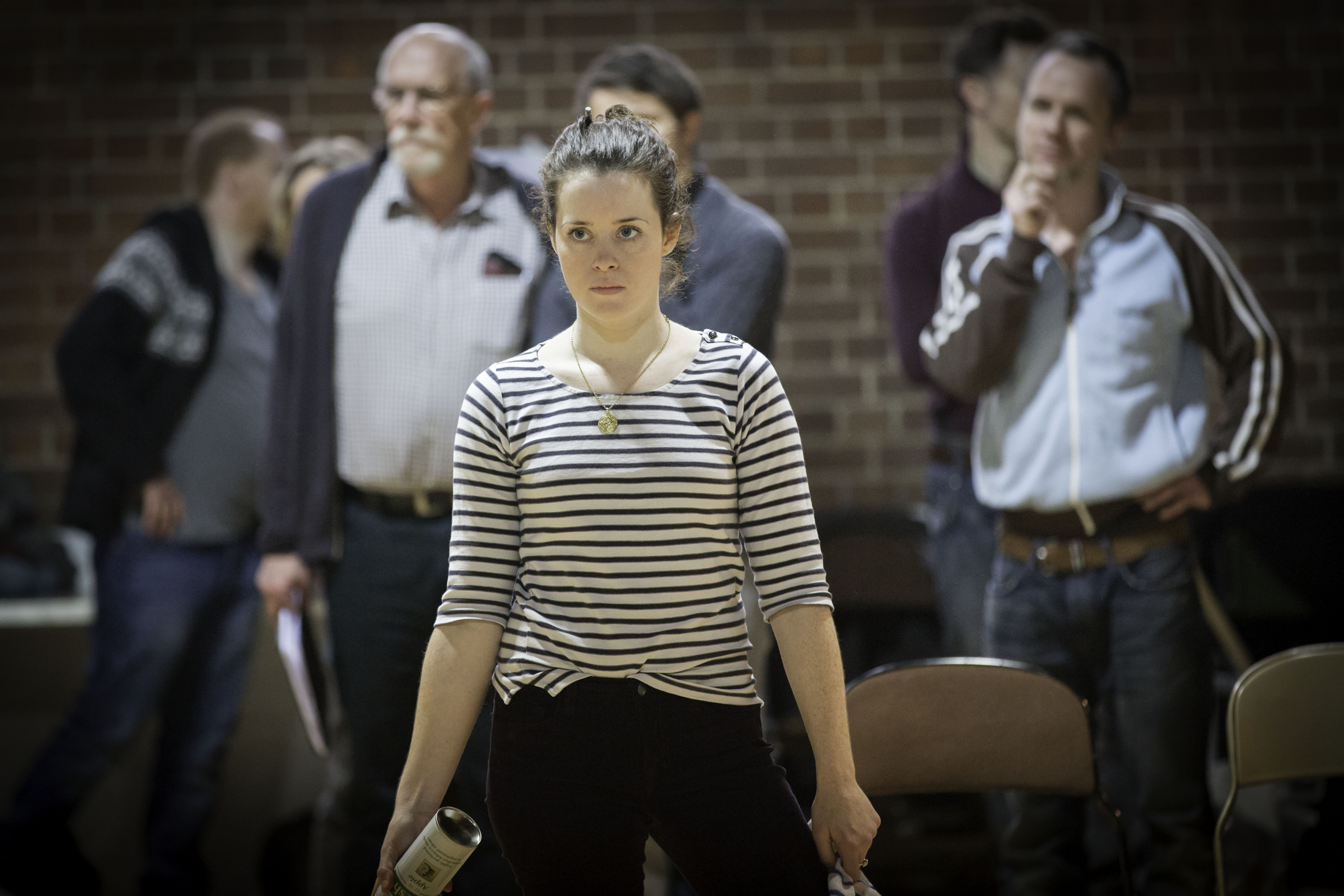A serious-looking woman with her hair tied back is captured standing indoors in front of a group of people. She is wearing a black-and-white striped shirt and black pants. In one hand, she holds a spray bottle, and in the other hand, a cloth, suggesting she might be performing or demonstrating something on stage. To her right is a folding chair with a brown seat and black trim. Behind her, at least six people are visible; the lighting focuses on the center, leaving the edges darker. Among the onlookers is an older man with glasses, a white beard, and a goatee. The backdrop consists of a brown brick wall, adding to the indoor setting's ambiance.